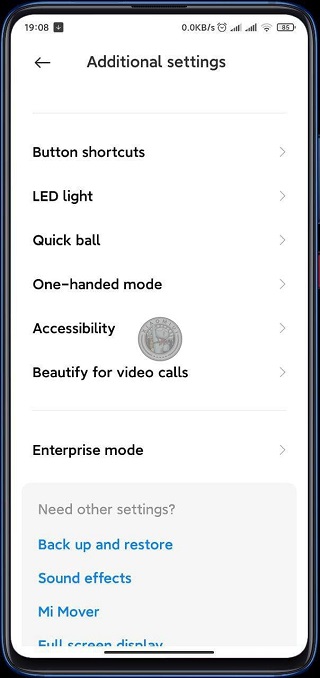The digital image displays the settings menu of a cell phone, organized in a detailed and structured manner. At the top of the screen, the time is shown in military format as "19:08." The status bar also features Wi-Fi signal bars, a battery icon indicating 85% charge, and an alarm clock symbol.

Just below the status bar, the title "Additional Settings" is prominently displayed in black, accompanied by a leftward arrow. The menu contains several options listed sequentially:

1. **Button Shortcuts**
2. **LED Light Option**
3. **Quick Ball**
4. **One-Handed Mode**
5. **Accessibility**
6. **Beautify for Video Calls**
7. **Enterprise Mode**

Further down, there are more options:
8. **Need Other Settings?** (accompanied by a question mark)
9. **Backup and Restore**
10. **Sound Effects**
11. **Mi Mover**
12. **Full-Screen Display**

The text for these options is styled in blue, ensuring they stand out against the background. Each option is formatted clearly for easy navigation and user interaction.